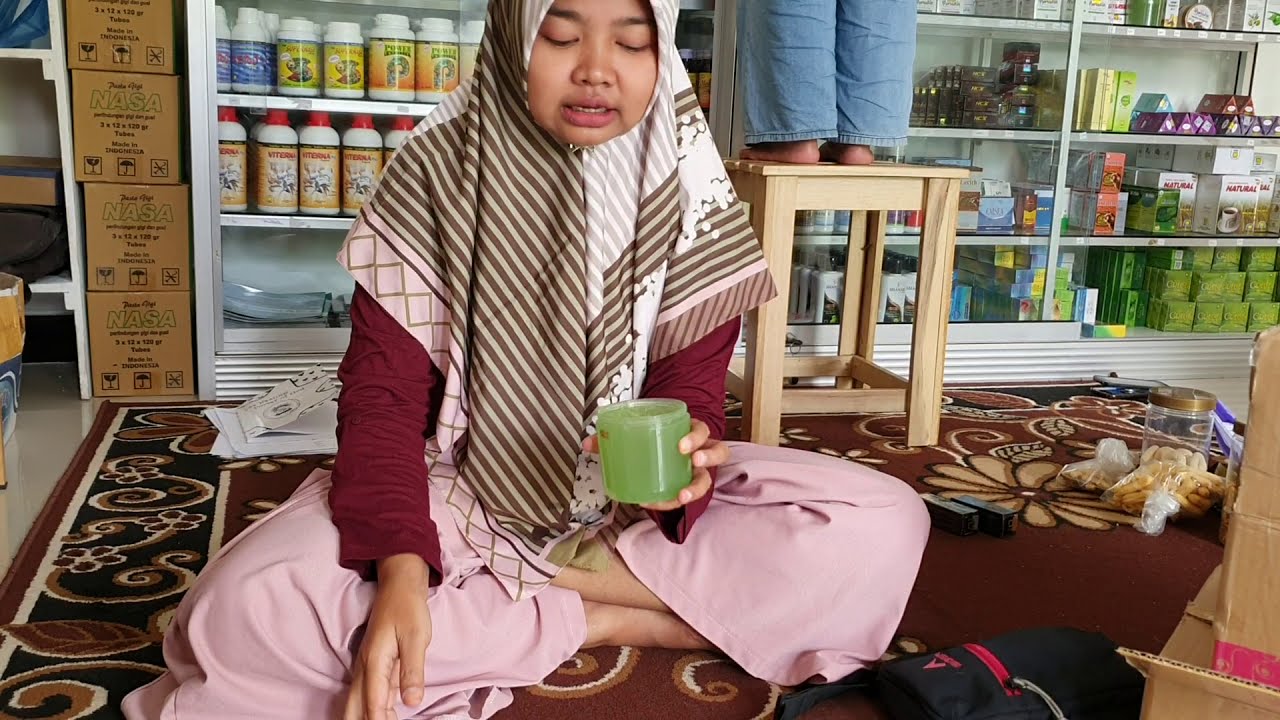The image portrays a young Asian lady seated cross-legged on a red carpet with a paisley print. She is dressed in loose pink pants and a maroon long-sleeved shirt. A distinctive hijab wraps around her head, featuring brown and white stripes on one side and gray and white stripes on the other. She is barefoot and holds an open green container in her right hand, gazing down at it, revealing the bottom of her teeth with her slightly open mouth. 

Behind her, a person stands barefoot on a wooden stool, donning long blue pants. The background is filled with an assortment of items, including a white shelving unit stocked with various bottles and boxes. To the left of the lady, boxes labeled NASA are piled atop each other. To the right, there are multiple glass cabinets filled with rows of items: the left cabinet has bottles with red and white caps, bearing different symbols, and the other cabinets are stocked with black, blue, purple, and green boxes arranged on three layers. The intricate details and array of objects suggest a busy, possibly medicinal environment.